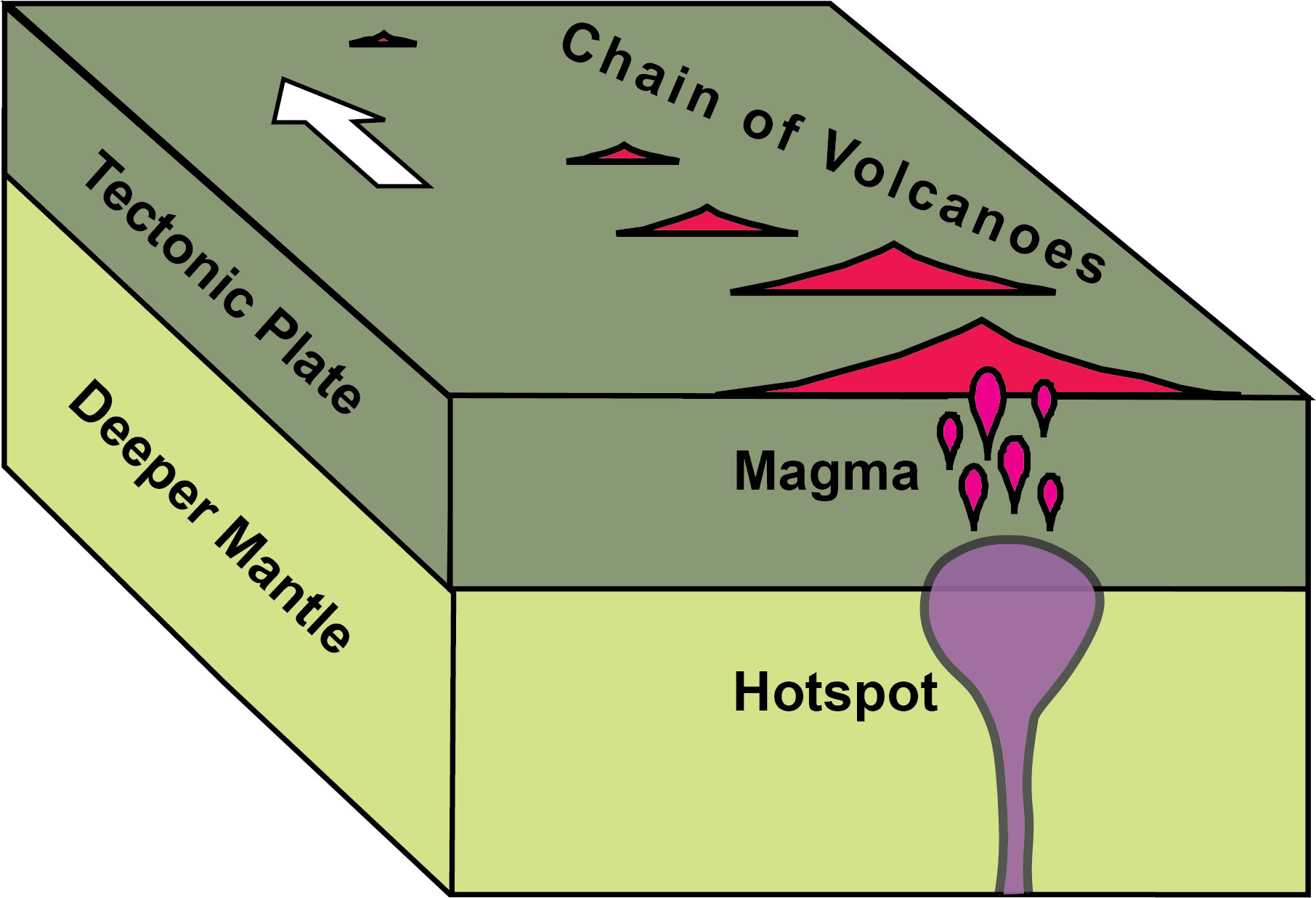This detailed illustration depicts the operation of a volcano within a 3D, slightly off-center, rectangular box. At the top of the image, a chain of volcanoes is represented by red triangles, with an arrow labeled "Chain of Volcanoes" pointing upwards. Below this chain lies the tectonic plates, shown in an olive color, indicating their movement. 

Underneath the tectonic plates resides a section labeled "Magma", colored purple with bright pink droplets indicating the magma's components. Beneath this, at the bottom of the box, a "Hot Spot" is depicted, which is connected to the "Deeper Mantle" in a light green shade. The detailed labels and color codes effectively illustrate the layered structure and dynamic processes of volcanic activity, making it an informative graphic suitable for educational purposes, perhaps in a museum exhibit.